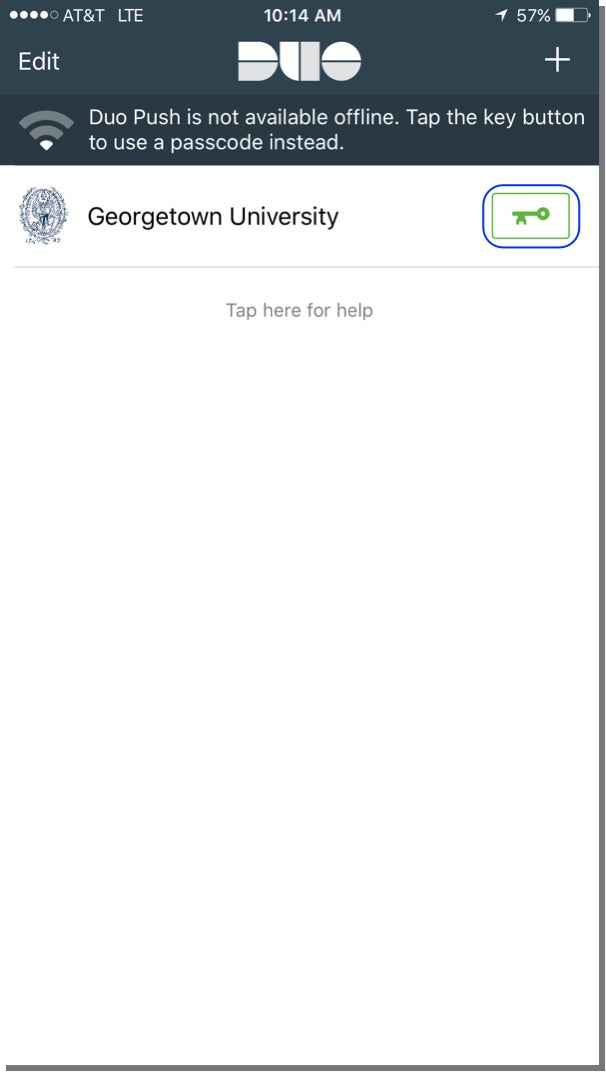The image is a screenshot taken from a smartphone displaying various interface elements. 

The top portion of the screenshot features the standard status bar icons: on the top-left corner, the network signal strength is indicated along with the service provider, AT&T, and the connection type, LTE. The top-center shows the current time, 10:14 AM. On the top-right, the battery icon indicates a 57% charge. The background of the status bar is dark.

Below the status bar, the main content of the screen revolves around the Duo Push application interface. The interface's header has the text "Duo," written in white, centrally aligned, with two icons at either side: "Edit" on the left and a "+" (plus) sign on the right. Underneath the header, a message reads, "Duo Push is not available offline. Tap the key button to use a passcode instead." To the left of this text is a Wi-Fi signal icon showing one bar out of three.

Below this header message is a section related to Georgetown University. The text, "Georgetown University," is prominently displayed in black on a white background, accompanied by the university's logo on the left. To the right of the university name, there is a green key icon surrounded by a blue circle, indicating a place to tap for additional functionality. Directly beneath this, in smaller text, it says, "Tap here for help," against a clean white background, possibly offering further assistance or support options.